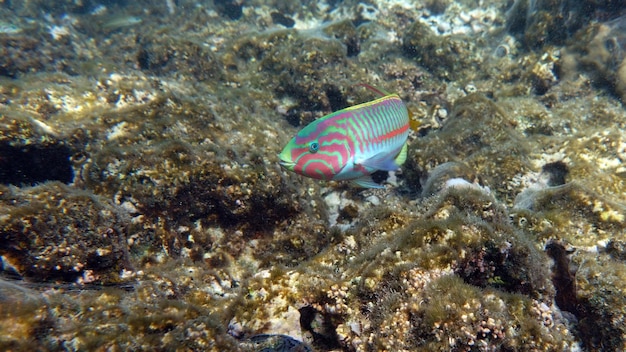This striking, modern underwater photograph captures a vividly colorful tropical fish centered amid a rocky, sea-bottom landscape that appears to be composed of volcanic material. The bottom terrain is adorned with patches of moss or seagrass, adding to the underwater environment. The fish's base color is a dynamic blend of lime green transitioning to yellow along its back and blue along its belly, creating a mesmerizing gradient. Prominent vertical red stripes cascade from the fish's dorsal side down to its belly, with an additional thick red stripe extending from behind the head to the tail. The fish also exhibits intricate red markings around its face. Its fins sport a deep, mystical blue hue. The vibrant and almost cartoon-like appearance of the fish stands out against the muted, whitish-green shades of the coral and algae background, making for an eye-catching and unique underwater scene.